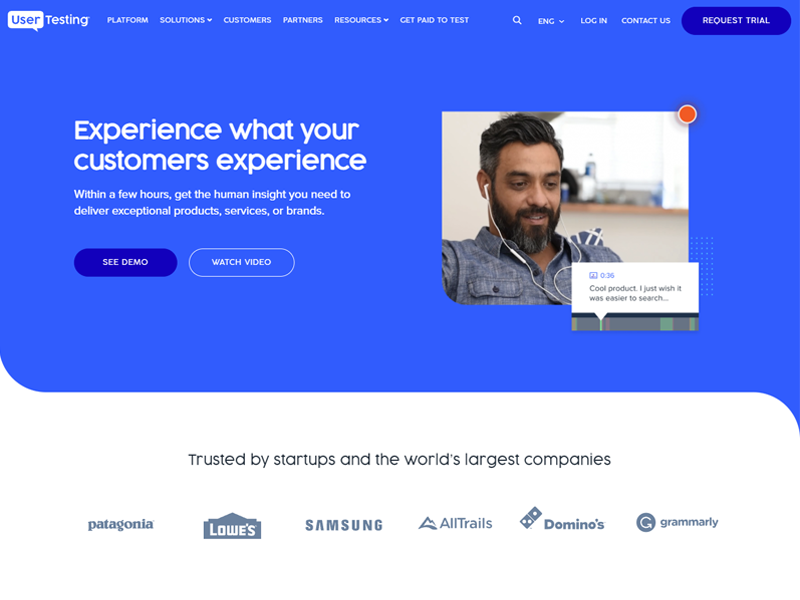The image depicts a brightly colored website primarily featuring shades of vivid blue. The layout includes a distinctive design element in the lower right-hand corner, where an image takes the form of a speech bubble, suggesting someone is communicating a message. 

At the top of the webpage, the navigation bar includes clickable options such as "Platform," "Solutions," "Customers," "Partners," and "Resources." Additionally, there are buttons for getting paid to test and requesting a trial, the latter in a prominent blue oval button located in the upper right corner. The header also features options for "Contact," "Login," and a language selector labeled "ENG English," indicating the availability of a dropdown menu for switching languages.

The main section of the page features the headline, "Experience what your customers experience within a few hours," accompanied by the subtext, "Get the human insight you need to deliver exceptional products, services, or brands." Directly beneath this text are buttons labeled "See Demo" and "Watch Video."

A large, central image showcases a man with a beard and mustache, black hair, and wired earphones. He appears to be intently focused on something, likely located off-screen, with a kitchen visible behind him, suggesting a home setting. 

An orange dot in the corner near him displays a quote: "Cost product I just wish it was easier to search." 

At the bottom, the website highlights its credibility by listing logos of prominent companies such as Patagonia, Lowe's, Samsung, AllTrails, Domino's, and Grammarly, accompanied by the statement "Trusted by startups and the world's largest companies."